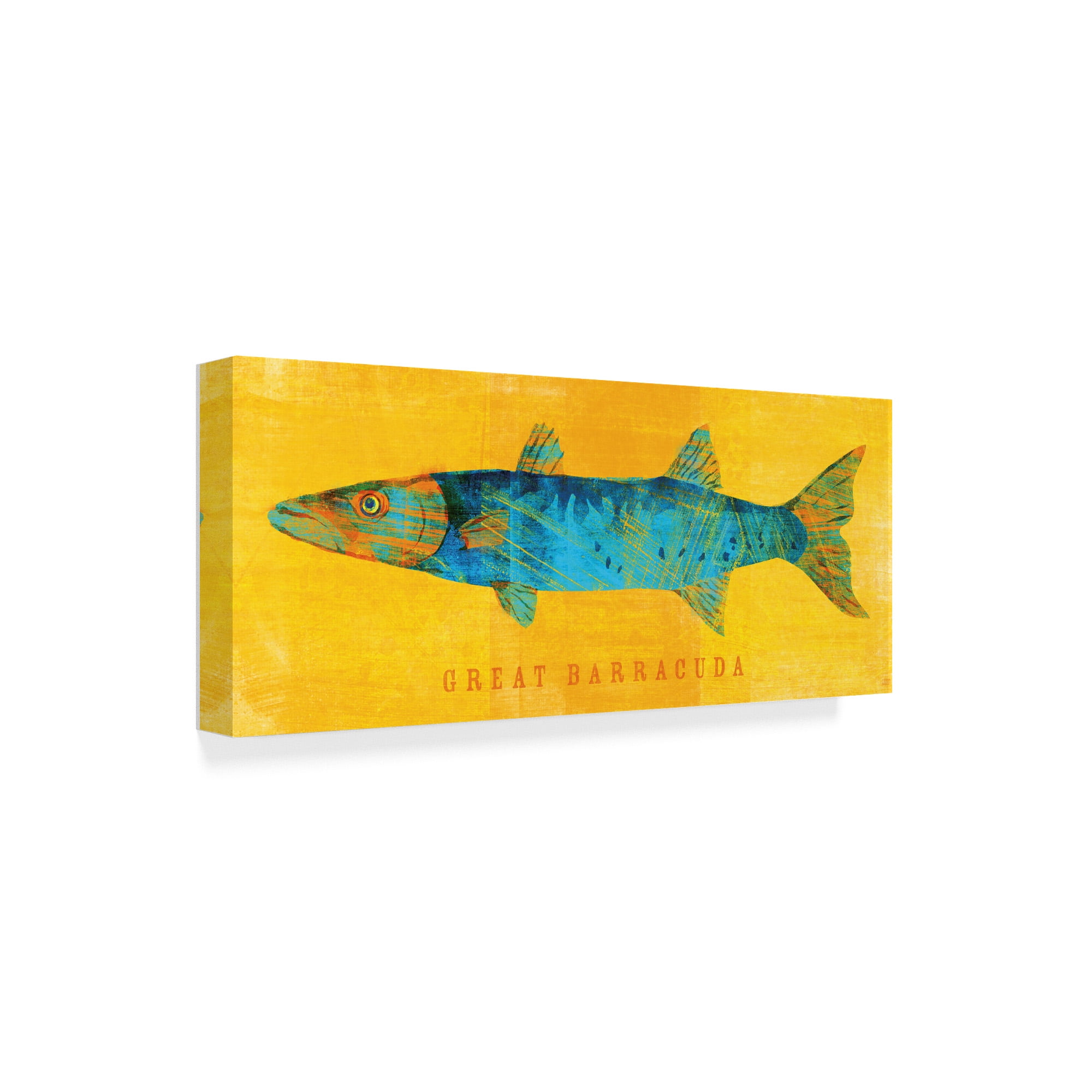This product photo showcases a rectangular canvas painting featuring a vibrant depiction of a Great Barracuda. The painting, which is slightly angled from left to right, reveals an artistic profile of the fish with a body predominantly painted in blue, accented with strokes of orange on the tail, face, and fins. The fish is set against a textured golden yellow background that adds depth and richness to the overall presentation. The canvas, likely stretched across a wood frame about an inch thick, includes a mix of hash marks and stripes across the colors, highlighting the intricate detailing of the artwork. Positioned at the bottom of the painting, in bold orange uppercase letters resembling the Times New Roman font, are the words "Great Barracuda." The photo itself is taken with a white backdrop and exhibits minimal shadowing, allowing the vivid colors of the canvas to stand out distinctly.